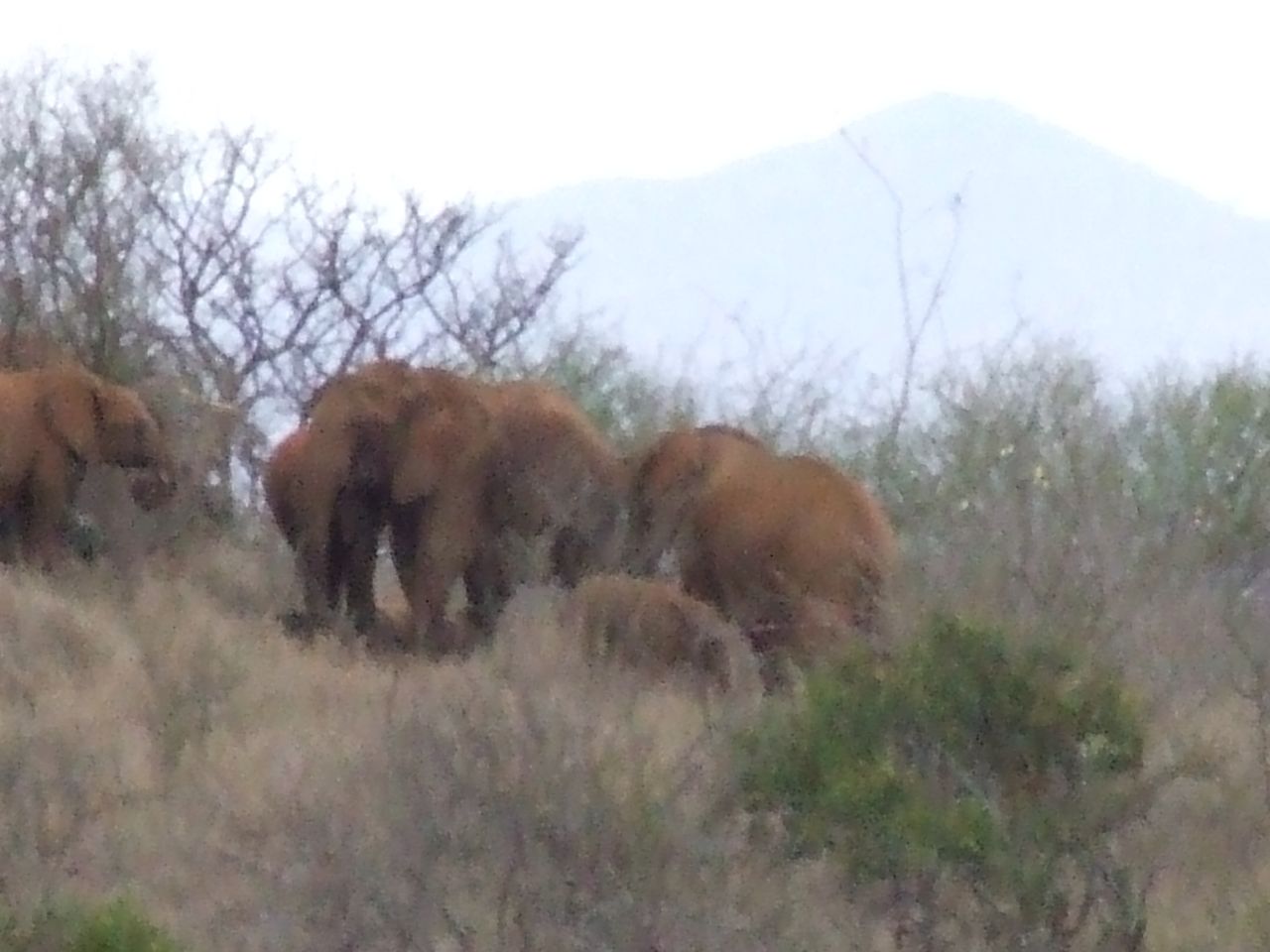This is a very blurry color photo of a group of five elephants in the wild, including four adults and one baby. In the foreground, you can see a field of bramble and high, brownish-green grass with patches of burnt grass. The elephants, all various shades of brown, are standing in front of a number of sparse trees. Some trees are barren while others have green leaves. Three adult elephants are in the center, with one adult elephant partially visible off to the side on the left. The baby, barely discernible, blends with the grayish-brown, almost dead-looking grass and is positioned near the adults. In the background, a foggy, sun-washed mountain, possibly Mount Kilimanjaro, adds to the scenic beauty of this presumed African landscape.